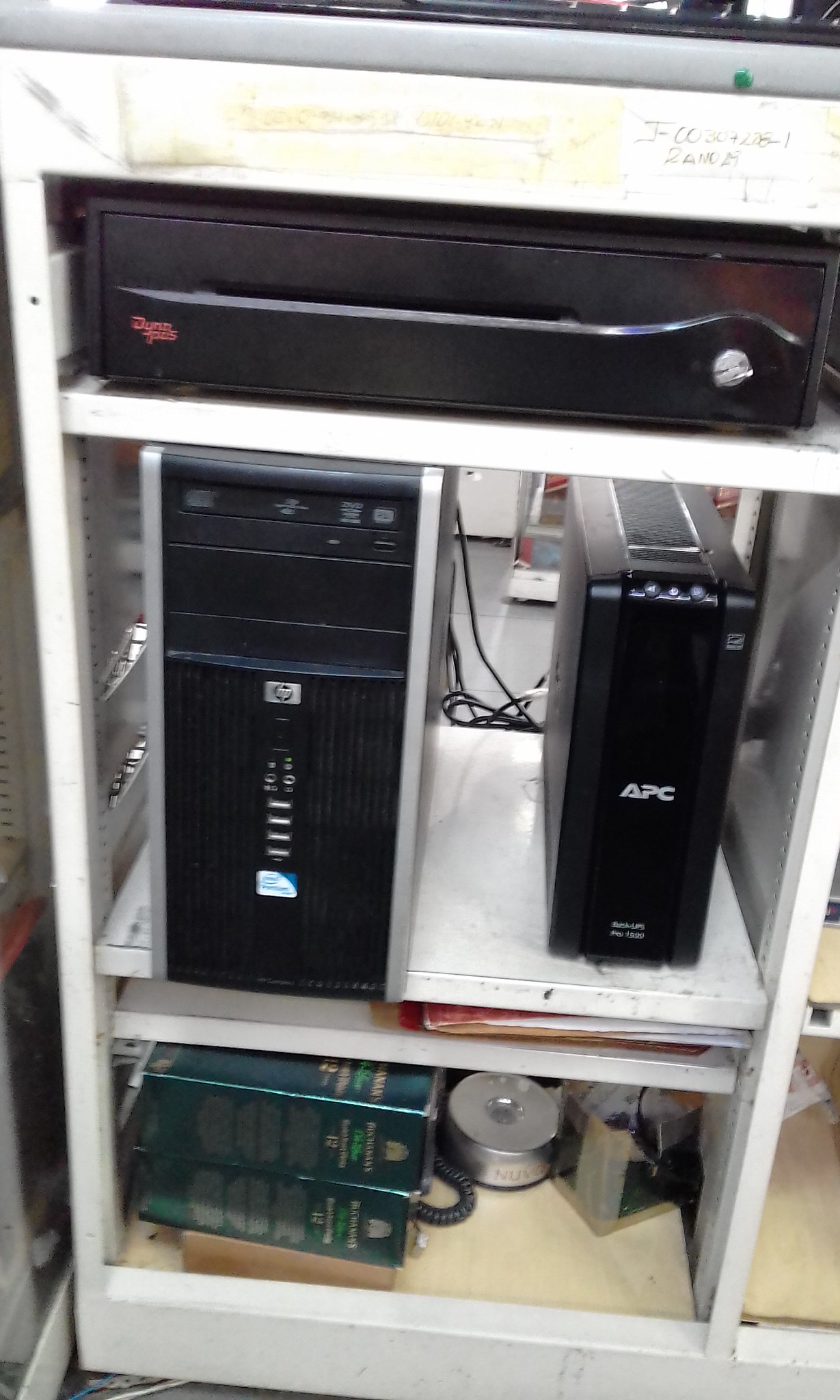In the image, we see a white metal computer cabinet that appears a bit aged and dinged up, with various objects neatly arranged on its shelves. At the bottom shelf, there are a few books, possibly a tool, and some green-colored boxes. The middle shelf houses two computer towers—one labeled as an APC and the other as an HPC—positioned near the center of the image. The top shelf contains what looks like a safe or a lock box. The cabinet itself is equipped with trays that might pull out, and numerous cords can be seen trailing behind the equipment. The setup, likely located in an indoor computer room or server area, displays a range of colors including black, white, gray, yellow, red, light blue, and green.